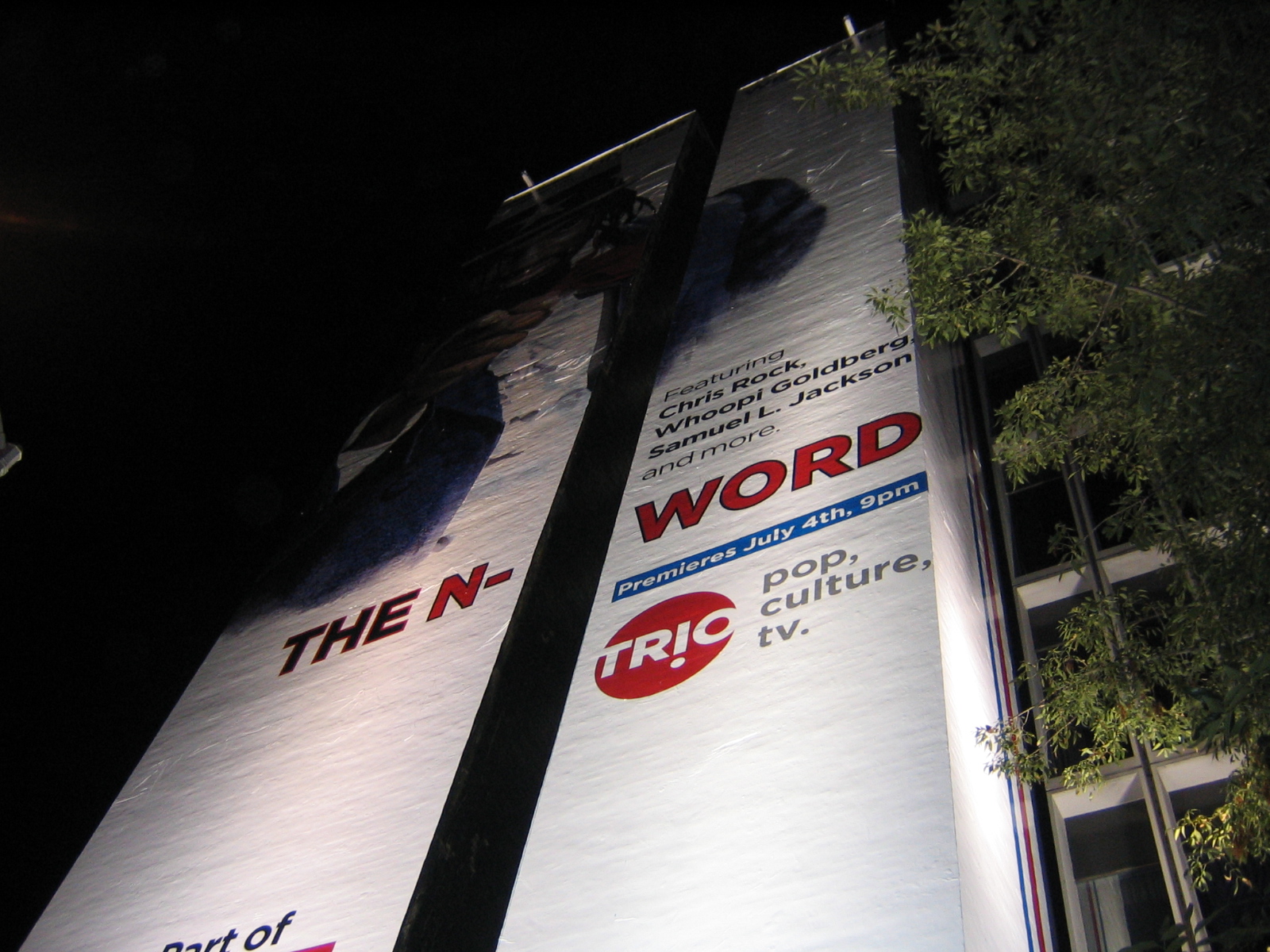The nighttime photograph showcases an enormous vertical billboard, approximately eight stories high, mounted against a gray office building with stacked rectangular windows. The billboard, with a pristine white background and a large black vertical line down its center, stands prominently illuminated, and a tree with green leaves is visible on its right side. 

The central focus of the billboard is the title "The N-Word"; "the" is in black, "N" is bold red, followed by a dash and "word" in black. Just below this title, it details the premiere date: "July 4th, 9 p.m." This special features Chris Rock, Whoopi Goldberg, Samuel L. Jackson, and more, and will air on Trio Pop Culture TV. The Trio logo, a distinctive red circle with white font, has the upside-down "I," and beneath it, the tagline "pop, culture, TV" aligned vertically in gray. There is also a graphic suggesting a figure holding or firing a weapon, spanning across the top of the billboard. This substantial and visibly prominent advertisement appears to be for a significant discussion or presentation on sensitive language in black history programming.